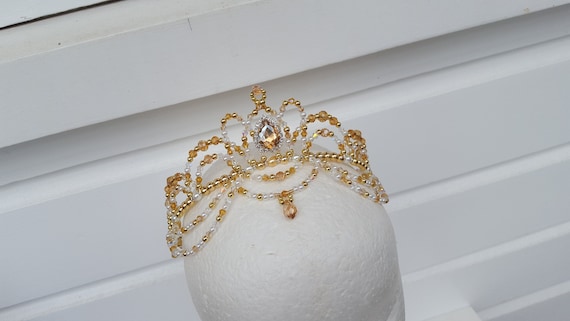The image captures a detailed and ornate tiara, resembling a crown, resting on a plaster cast mannequin head. The tiara is intricately designed with a combination of gold and pearl beads, and features multiple loops of gold throughout its structure. A large, shiny silver jewel is prominently positioned at the center, just above the headband, surrounded by semi-circular layers that enhance its regal appearance. The backdrop consists of white wooden panels arranged diagonally, giving the setting a unique aesthetic. The light-colored, slotted door in the background, resembling a garage door, creates a stark contrast to the elegant tiara displayed in the foreground. The photograph is taken in landscape mode, emphasizing the tiara's luxurious details against the unconventional and clean background.